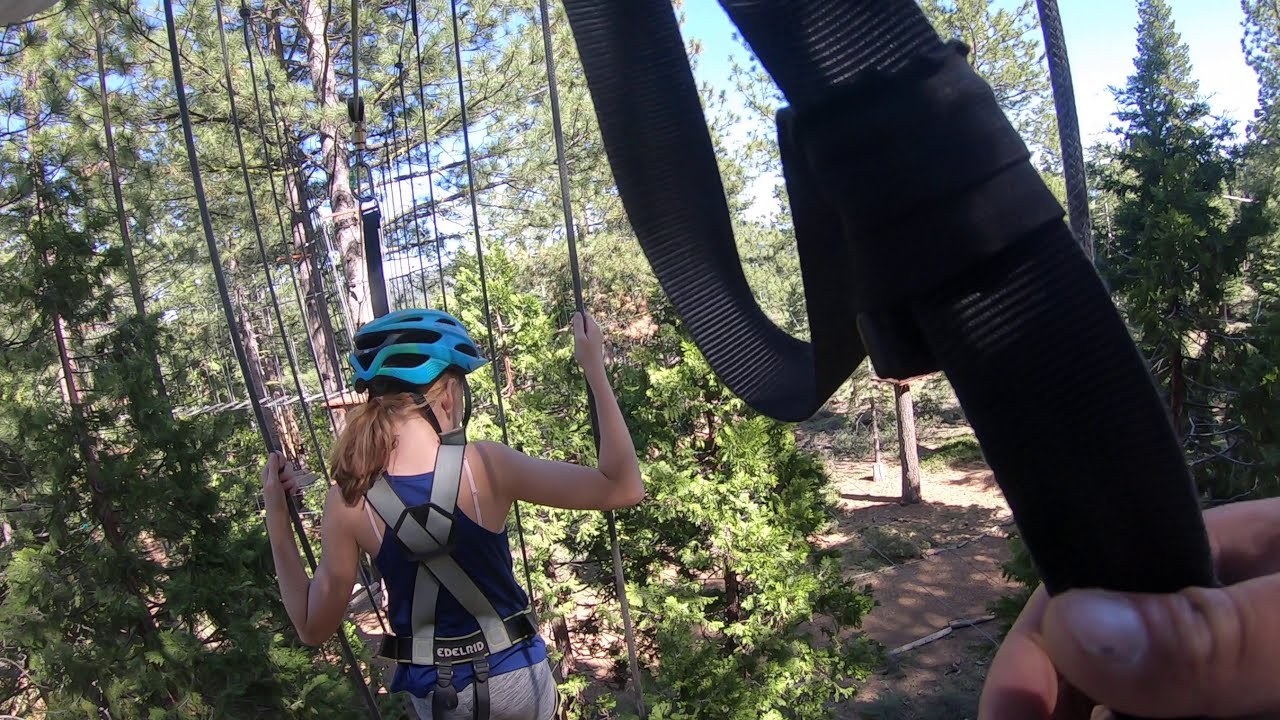The image captures an exhilarating scene of people ziplining through a lush forested area under a bright daytime sky dotted with white clouds. In the center of the image, two individuals are ziplining close together. The person in the foreground is partially visible, with their right hand gripping a sturdy black strap. Just in front of them, a woman is prominently featured, wearing a blue sleeveless tank top and gray shorts, secured with a gray harness that crisscrosses her torso. She sports a blue helmet with black chin straps and appears to be firmly holding onto various ropes attached to a black canvas harness, which is hooked onto a cable above her head. The forest below is densely green, with patches of visible dirt, adding to the adventurous ambiance of the ziplining activity.